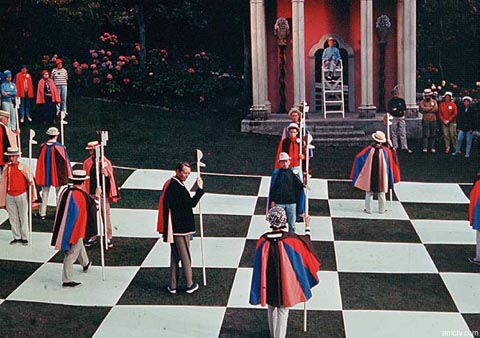The image depicts a human chess scene set on a black and white checkered ground at a diagonal angle. Participants stand on the squares, adorned in vibrant red, blue, pink, and black capes, paired with white pants, and some are holding white staffs. Surrounding the scene are lush areas with pink flowers and greenery, as well as white columns framing a reddish-colored building. Observers are present on both the left and right sides, with one individual seen on a ladder. Despite being daytime, the background is somewhat dark, reminiscent of an aesthetic from the 1960s.